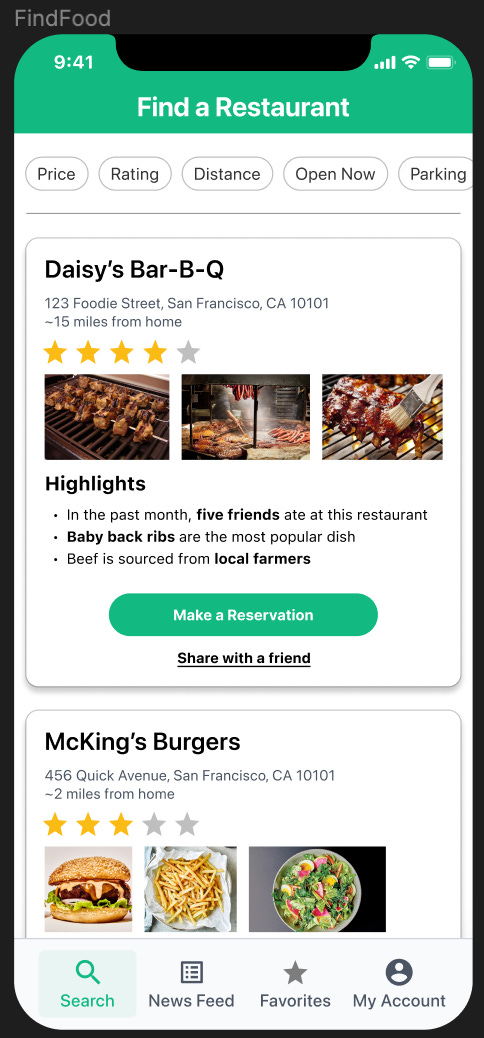A screenshot of an iPhone mobile application is displayed, showcasing a web-like interface focused on food discovery. The screen has black edges at the top and bottom, typical of an iPhone design. At the very top, a green status bar displays the time as 9:41 on the left side, with icons indicating full mobile reception, full Wi-Fi strength, and a fully charged battery on the right.

The app interface header reads "Find Food" in the upper left-hand corner. Beneath this, a green band runs across the top. The middle section prominently displays a search function labeled "Find a Restaurant," accompanied by various search filters such as pricing, ratings, distance, "open now," and parking options in white text on a black background.

Two restaurant entries are featured below. The first entry is for "Daisy's Bar BQ" located in Newmarket Square, San Francisco, 15 miles from the user's home. It has a four-star rating and includes three images showcasing barbecued meats. Highlights note that five friends have visited this restaurant in the past month, the baby back ribs are the most popular dish, and the beef is sourced from local farmers. There is a prominent green "Make a Reservation" button and an underlined "Share with a Friend" option in black.

The second entry features "The King's Burgers," also in San Francisco, but just 2 miles from home with a three-star rating. The accompanying image shows a burger, fries, and a salad. 

At the bottom of the screen, green and white navigation options are labeled "Search," "Newsfeed," "Favourites," and "My Account."